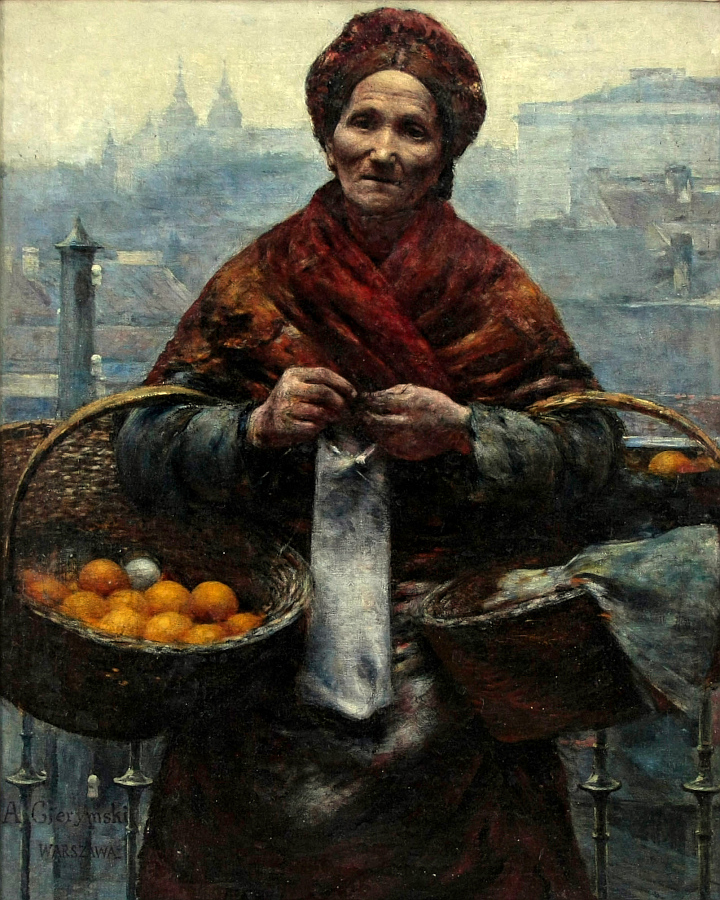This detailed painting depicts an elderly woman from a vintage era, standing prominently in the foreground against a backdrop of a cityscape with buildings, steeples, and possibly palaces with towers. The sky is a yellowish-gray, enhancing the historic ambiance. The woman, characterized by the deep wrinkles on her face, wears a traditional dark gray dress with frayed sleeves and a reddish-brown shawl draped around her shoulders and neck. She dons a brown headdress that adds to her antique appearance. Leaning on an ornate wrought iron fence, she holds two baskets: the one in her left arm contains tangerines and a white orb, possibly an egg, while the right arm's basket is covered with a gray cloth, concealing its contents. Additionally, she clasps a small white cloth bag in her hands. It is a bright, sunny day, lending clarity and vividness to the scene.